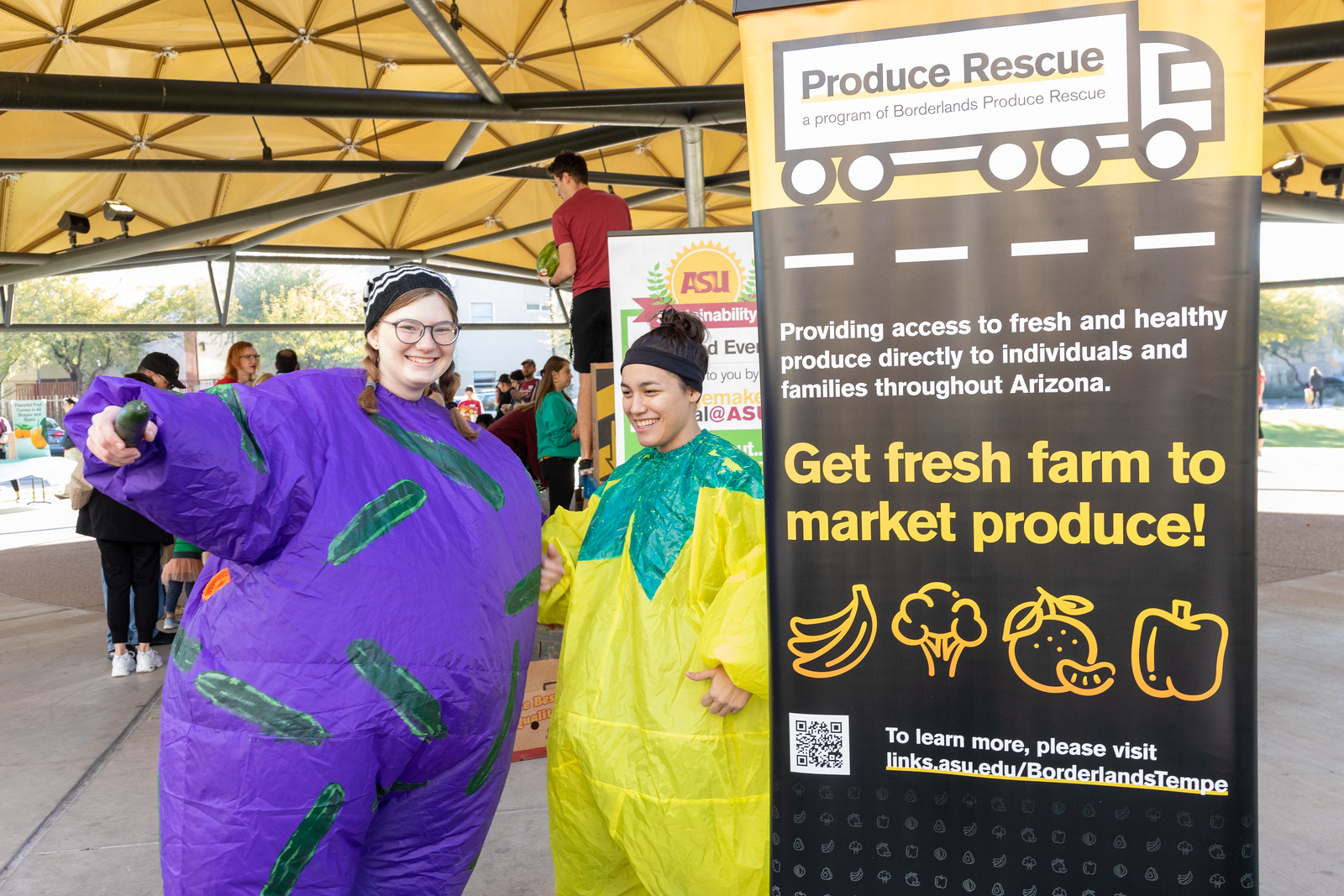In the vibrant scene under a yellow pavilion, two women in colorful inflatable costumes stand cheerfully beside a sign. The woman on the left, a redhead with dark-framed glasses and a black and white beanie, wears a purple suit adorned with what appear to be green vegetables and holds a cucumber in her right hand. Her hair is styled in two short braids. The woman on the right has dark hair tied in a bun and is clad in a yellow and green costume, complemented by a black headband. They are positioned by a vinyl sign that reads, "Produce Rescue, a program of Borderlands Produce Rescue," depicted within a cartoon truck on a road. Below this, the sign states, "Providing access to fresh and healthy produce directly to individuals and families throughout Arizona," and further encourages, "Get fresh farm-to-market produce!" with illustrations of various fruits and vegetables. A QR code at the bottom prompts viewers to visit links.asu.edu/BorderlandsTempe for more information. The background reveals a setting with trees and parkland, where other people are engaged in festival activities, including a man on a step ladder. The lively atmosphere suggests a community event aimed at promoting fresh produce and healthy eating.